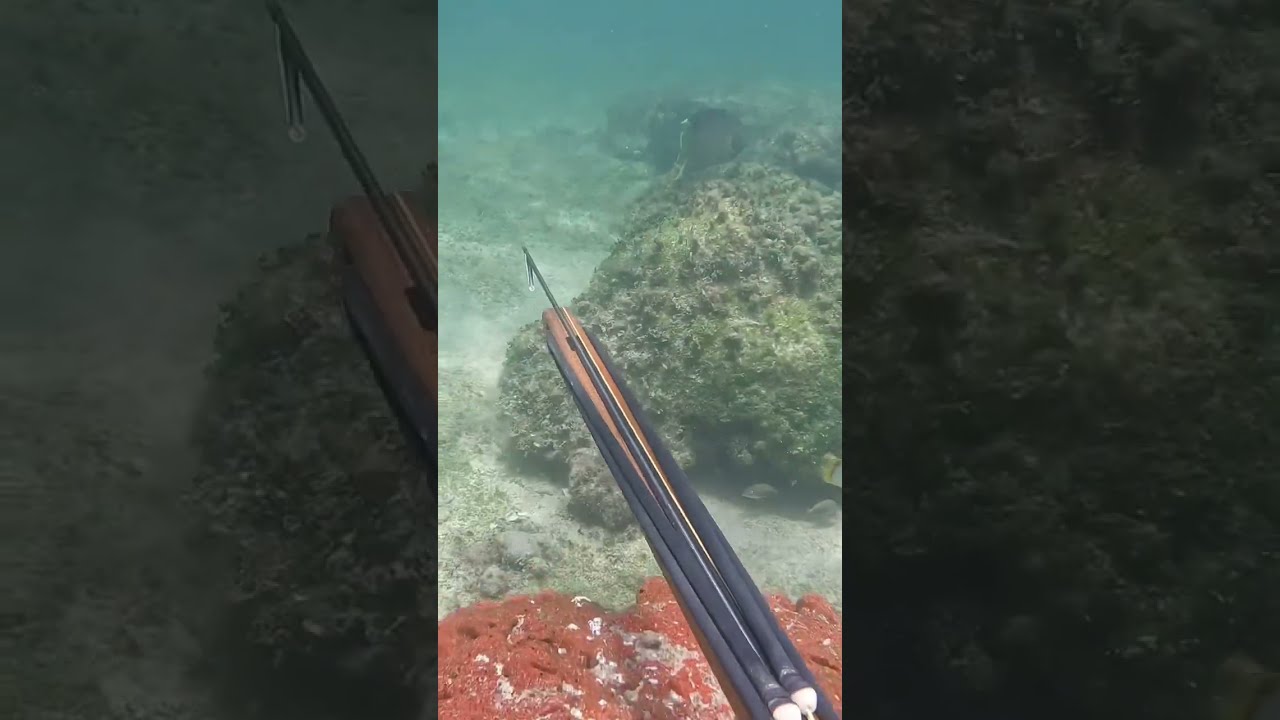The image is an underwater photograph taken near the ocean floor, capturing an active spear fishing scene in daytime with very clear lighting. The main focus is a wooden spear with a metal tip, equipped with a rubber tie mechanism for shooting. The spear is angled from the bottom right to the upper left, emerging from the lower right-hand corner. Below that, a vibrant, reddish-orange rock or coral reef stretches from left to right. Behind this, larger green and gray reefs rise up, creating a layered aquatic landscape. 

The water around the reefs is clear at the bottom, transitioning to a murky bluish-green hue towards the top. In the background, a faintly visible sea snake can be seen swimming, although it's difficult to make out in detail. The photo is divided into three sections: the central part features the spear and reefs, while the left and right sections are darker, enlarged segments of the central image, highlighting the top of the harpoon on the left and the gray-green coral on the right.